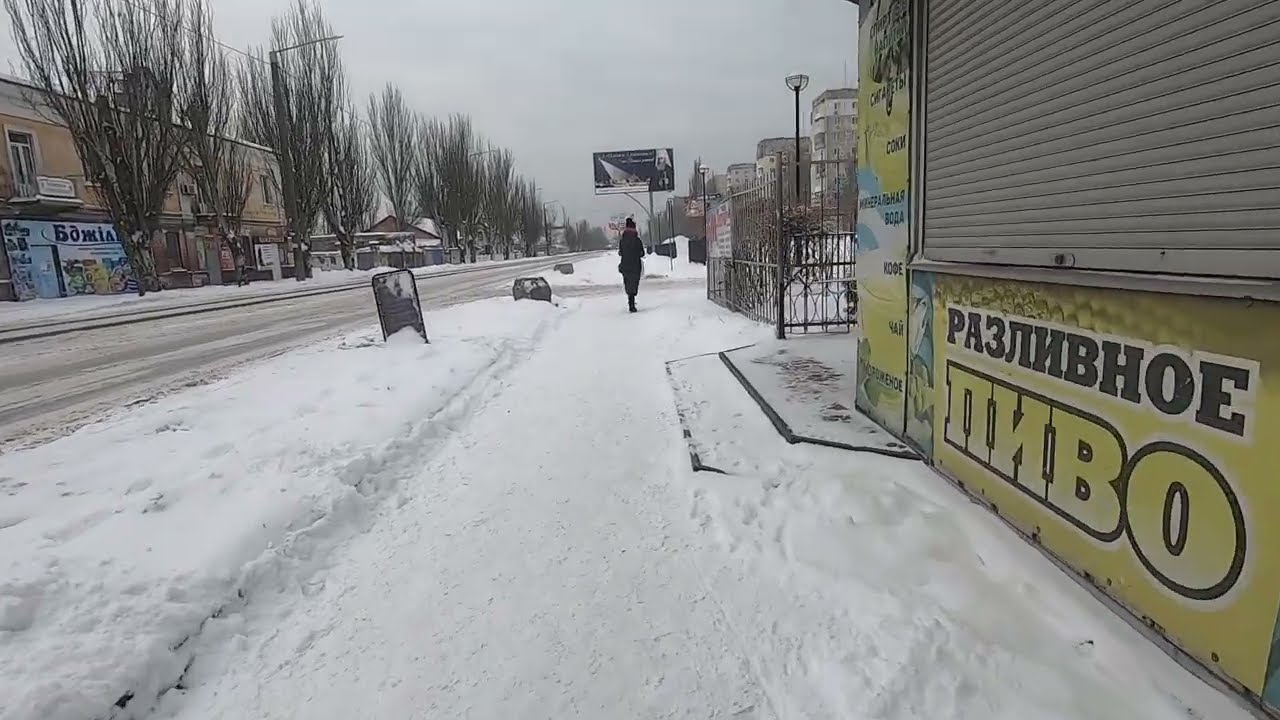The image depicts a snowy city street in what appears to be a Russian city. The viewer's perspective is from a sidewalk that extends from the bottom center of the frame towards the horizon line. To the left, the snow-covered street runs parallel to the sidewalk, bordered by a row of trees and several buildings. The right side of the image features a closed shop stall with a large yellow sign displaying text in what looks like Russian characters, possibly advertising items like lemonade. A black wrought iron fence appears next to the shop. In the distance, a person dressed in all black, including a black jacket and a hat or beanie, walks away from the camera. The overall scene is set in winter, with compacted snow covering the sidewalk and visibly iced-up roads. Farther in the background, various billboards and signs in Russian dot the urban landscape, along with tall buildings lining both sides of the street.